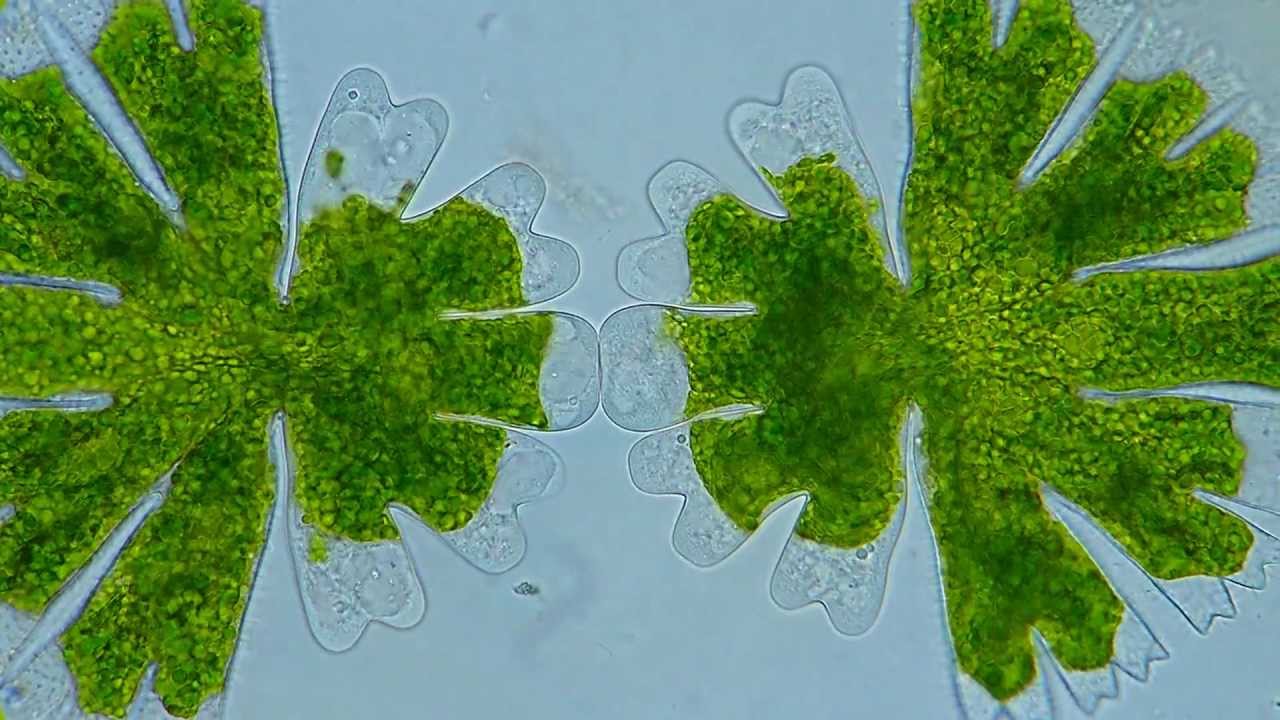A high-resolution microscopic image revealing a fascinating gelatinous structure, possibly a biological specimen. Two leaf-like formations dominate the scene, with a greenish central core and radiating extensions. These extensions appear to mirror each other, resembling twin symmetrical shapes. The texture suggests a soft, pliable material, while the background contrasts with a serene bluish hue.